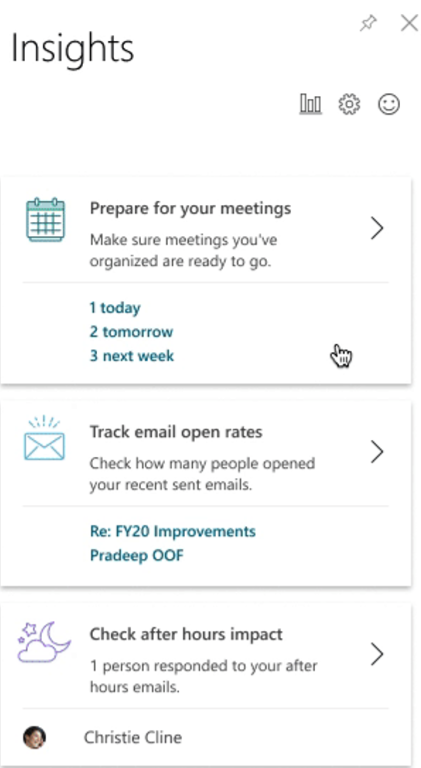At the top of the image, "Insights" is prominently displayed in large, black text. To the right, there are three vertical columns, reminiscent of skyscrapers. Adjacent to these columns, a small settings tool icon and a little happy smiley face are visible. Above these, there are icons for a pin and an X.

The lower section of the image is divided into three distinct parts:

1. The first section features a calendar icon and a message: "Prepare for your meetings. Make sure meetings you've organized are ready to go."
2. The second section displays an envelope icon next to the text: "Track email open rates. Check how many people opened your recently sent emails."
3. The third section shows a cluster of stars, a cloud, and a moon icon alongside the text: "Check after hours impact. One person responded to your after-hours emails."

At the very bottom, there is an icon of a person's head accompanied by the name "Christy Klein, C-L-I-N-E."